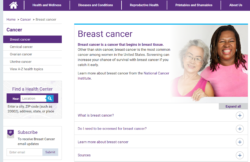The image features a digital screen focused on breast cancer information. At the top, a wide purple banner displays various navigation options. On the left side, a vertical column presents different selectable choices, with 'Cancer' highlighted in purple at the top of the list. Below this section, an option is visible, possibly indicating "Find a Health Career" or "Find a Health Center," providing a search functionality.

Occupying roughly one third of the screen, the page title "Breast Cancer" is prominently displayed in large, bold type. The visual content depicts two women; the older woman on the left is wearing a pink tank top, while the younger woman on the right is dressed in a pink t-shirt. The older woman’s hand is extended and curved as though holding an invisible sign, creating a notable 3D effect. This attention to detail emphasizes the human aspect of the breast cancer topic being presented.